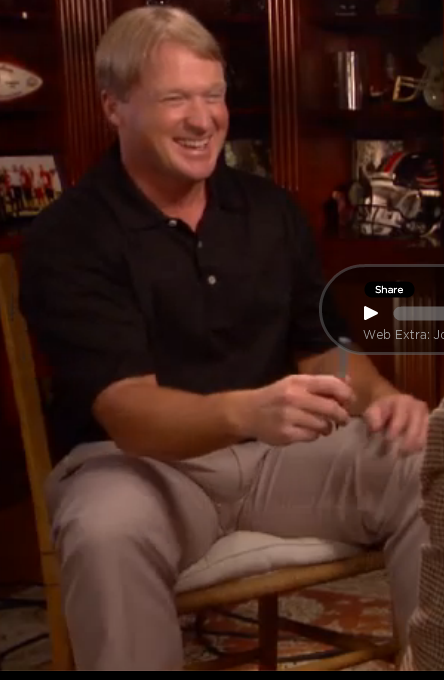This detailed color photograph captures a man with short blonde hair, seated on a brown wooden chair with a white cushion, which is only partially visible. He is dressed in a casual short-sleeve black button-down shirt and beige pants, and he appears to be smiling or laughing as he looks to his left. His right arm is raised slightly and bent at the elbow, holding what seems to be a pen. His left hand rests on his knee. The image appears to have been taken from a video, as evidenced by the time bar, share icon, and a play button labeled "WebExtra" on the right side of the frame. Behind the man, there is a brown wooden bookshelf filled with sports memorabilia, photographs, and a football helmet. The floor features a red and white oriental carpet, adding warmth to the cozy den setting.